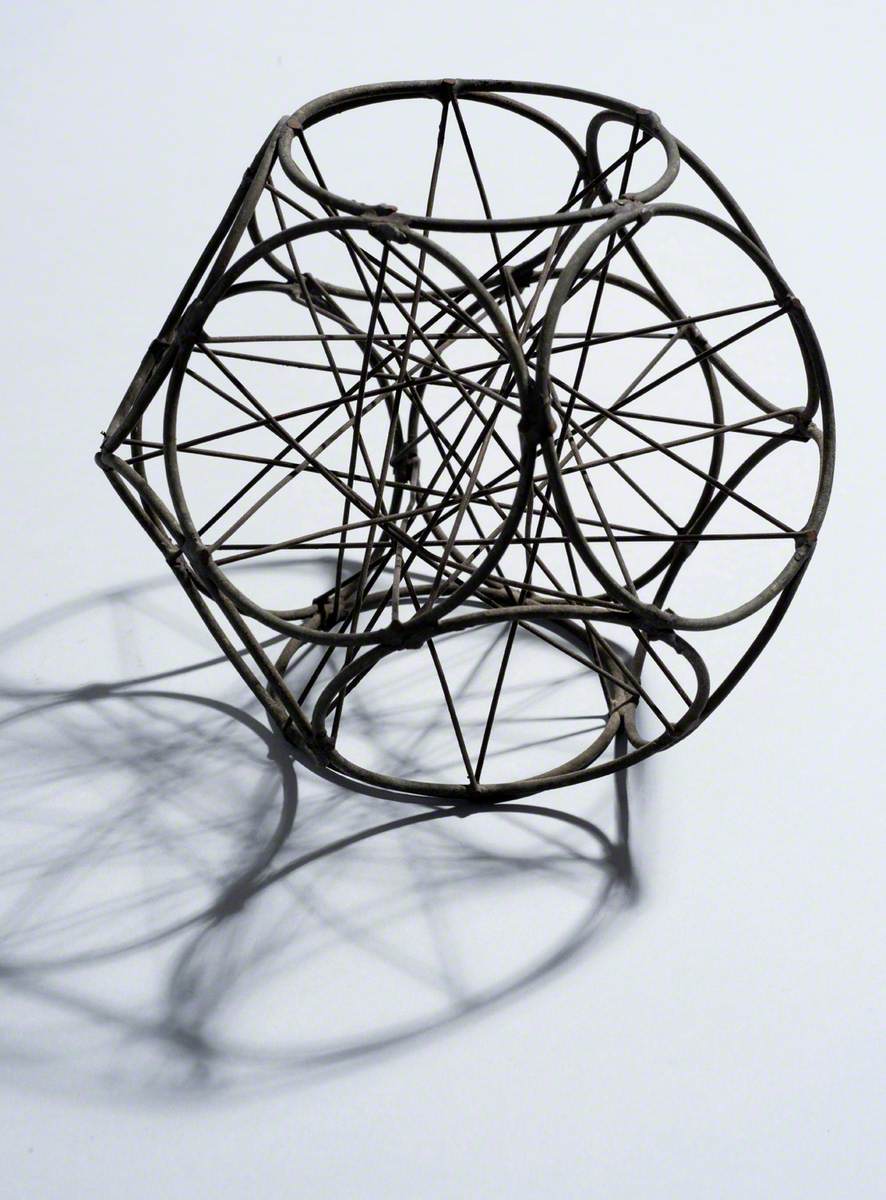The image features an abstract, intricate metal sphere sculpture composed of interlinked circular elements. These metal circles are meticulously welded or bolted together, creating a complex dodecahedron-like structure. Connecting the circles, a web of metal rods weaves through the interior, forming an interconnected lattice that adds depth and complexity. The sculpture appears black or dark-colored, standing out against a stark white background. It is carefully lit from above, casting a discernible shadow on the white tabletop, which emphasizes the delicate and artistic nature of the piece. This unique home decoration combines industrial materials with an abstract, almost chaotic design, making it an eye-catching artistic element.